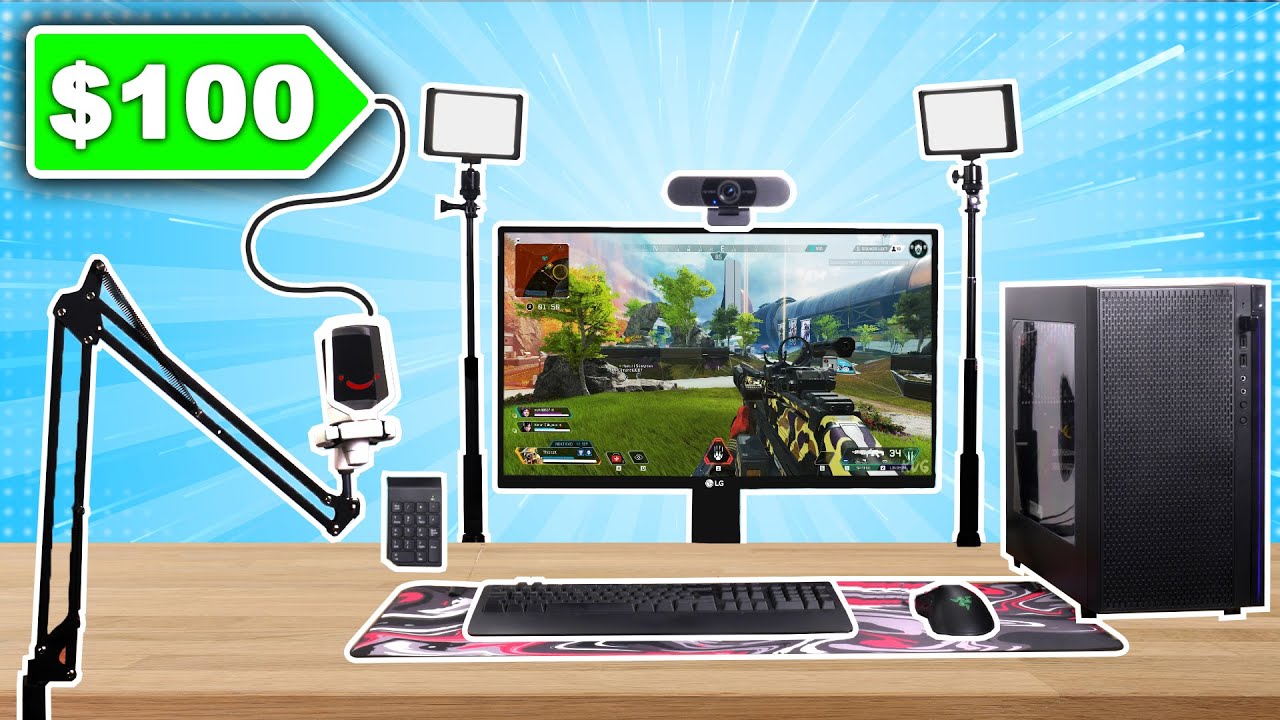The image depicts a detailed computer setup on a brown wooden desk. Central to the setup is an LG monitor displaying a shooting game, identifiable by a gun pointed within the game's backdrop. Clipped to the top of the monitor is a webcam, and it is flanked by two selfie sticks holding cell phones on either side. A pair of computer lights are also present on the desk. The keyboard and wireless mouse are positioned on a large mouse pad, with a nearby microphone stand featuring an angular design and a microphone at its end, attached to the desk. 

Additionally, the computer tower with a glass side allows a clear view of its interior components, and a USB stick is protruding from one of its ports. Other items on the desk include a large speaker, a smaller mini speaker, and what appears to be a remote control or electronic device on the left side. The setup is framed against a vibrant blue background with glowing dots. Notably, a green price tag with white text indicating "$100" is attached to the microphone stand, adding a prominent promotional detail to the image.